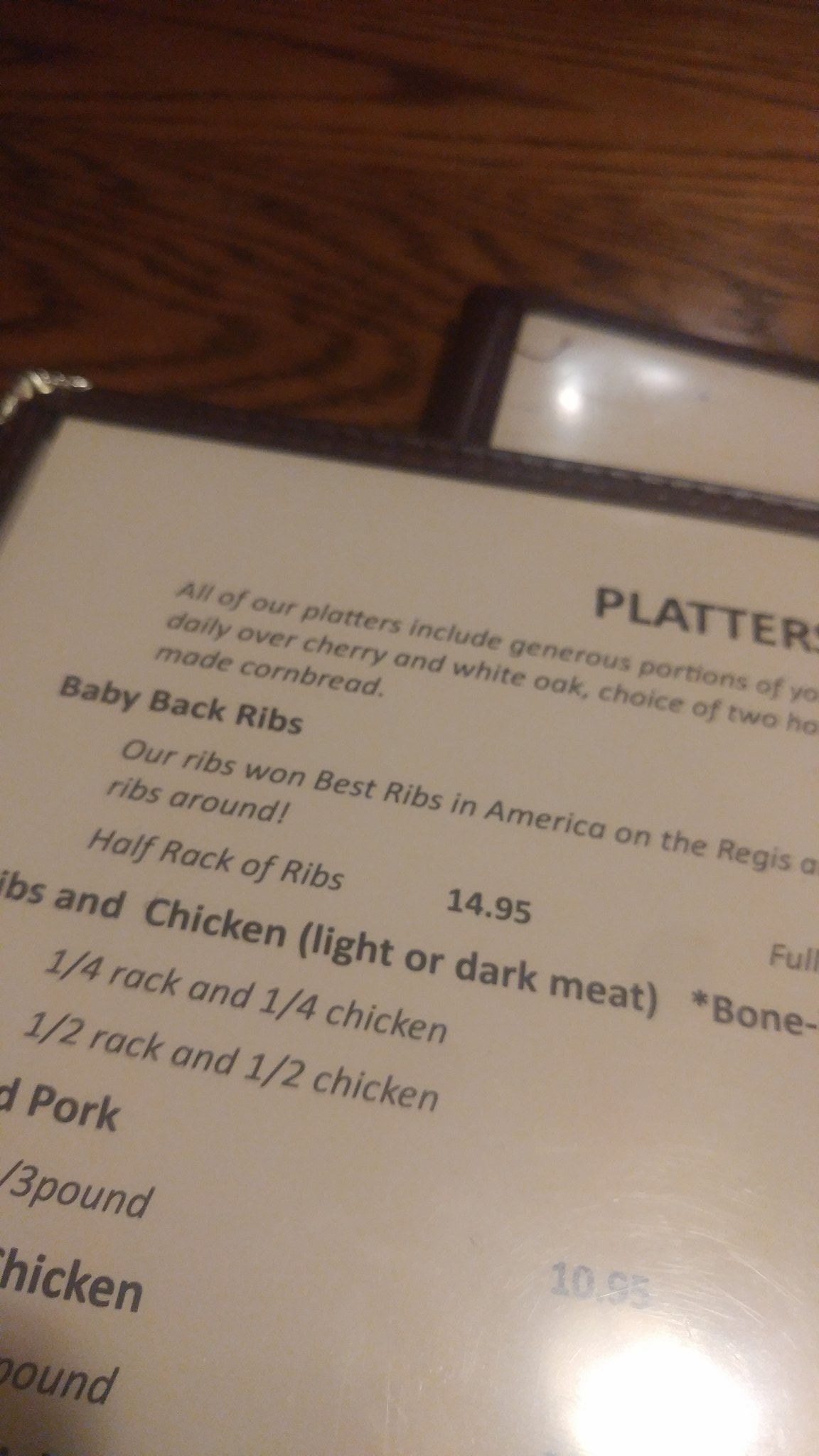This image reveals the upper left section of a restaurant menu. At the top, in bold black text, the word "Platter" is prominently displayed. Beneath this heading, a description in smaller text informs us that "All of our platters include generous portions of...," suggesting that the detailed list of items continues beyond the visible portion of the photograph.

Further down, the text mentions, "daily over cherry and white oak," hinting at a preparation method, followed by "choice of two." Additionally, the phrase "made cornbread" is discernible.

In bold black text, the item "Baby Back Ribs" is clearly labeled, and in lighter text, it is noted that these ribs "won Best Ribs in America on the Regis." The line continues with "Ribs Around," which appears cut off.

The menu lists "Half Rack of Ribs," priced at $14.95. Below that, the choice of "Chicken - Light or Dark Meat" is offered, with the word "bone" nearby. The options "Fourth Rack" and "Fourth Chicken" are present, followed by "Half Rack and Half Chicken."

The next bold heading is "Pork," below which only the words "three pound" are visible before the text cuts off. Nearby, "Chicken" is also mentioned.

In the lower right part of the menu section, the number "10.53" is visible. A bright, roughly two-inch wide circle of white light, presumably from an unseen light source, partially obscures this area. 

In the background, another menu can be seen directly beneath the primary one, adding depth to the image.